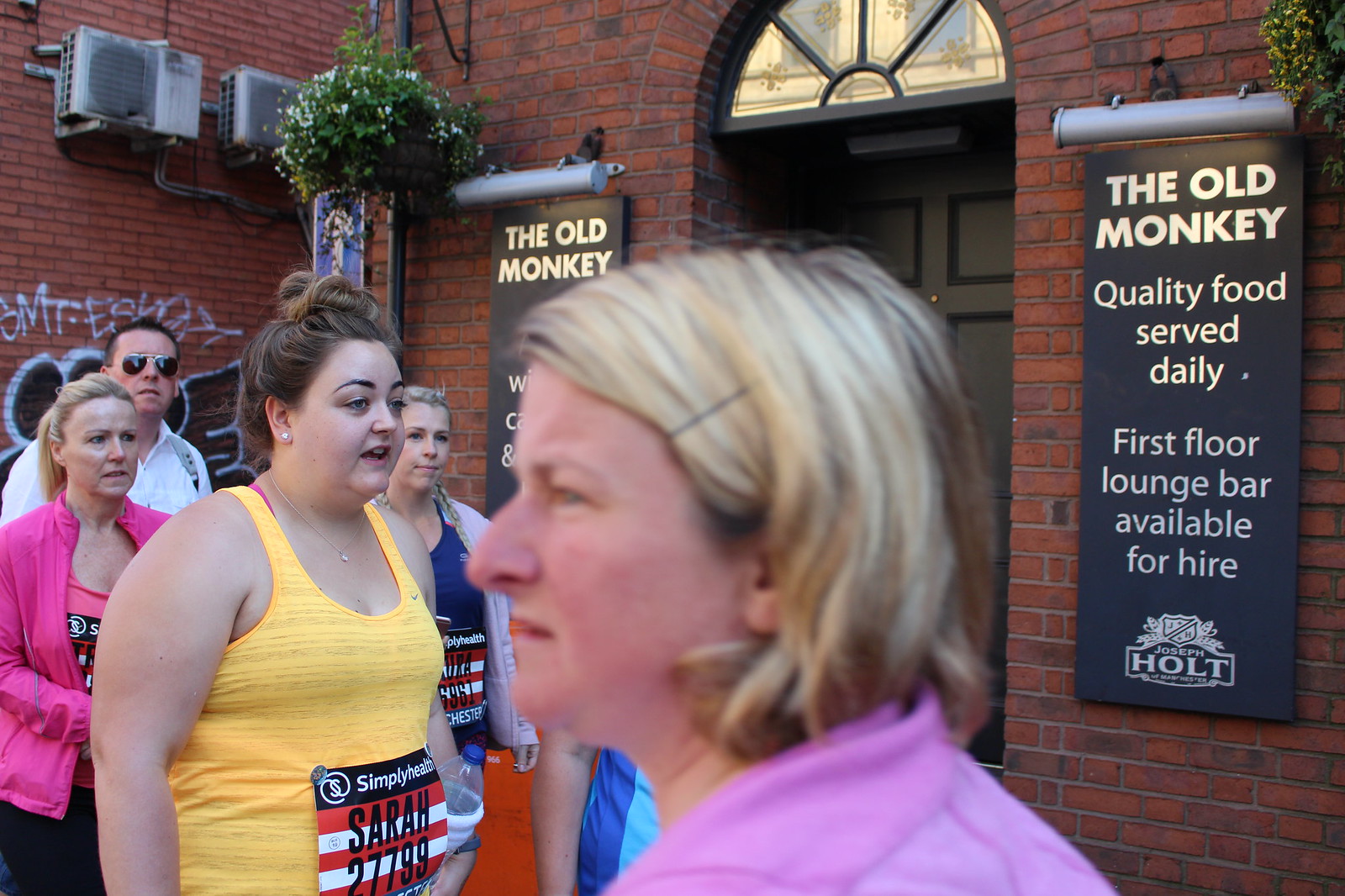This image captures a group of marathon participants standing outside a restaurant named "The Old Monkey," which features a traditional red brick exterior and a black door with a semi-circular window above it. Prominently displayed on either side of the door are banners that read "The Old Monkey, Quality Food Served Daily, First Floor Lounge Bar Available for Hire." A logo at the bottom of the banner references "Joseph Holt." 

In the foreground, a slightly out-of-focus woman with shorter blonde hair is dressed in a pink sweater. To her left stands an overweight woman wearing a yellow tank top and a race bib labeled "Simply Health," with the name "Sarah" and the number "27799." This suggests she is a marathon participant. Supporting this are two more female runners in the background, also sporting race bibs. Behind them, a gentleman can be seen, along with some graffiti on the building's brick wall. The scene is bustling with activity and provides a snapshot of marathon runners possibly taking a break or finishing their event near the restaurant.